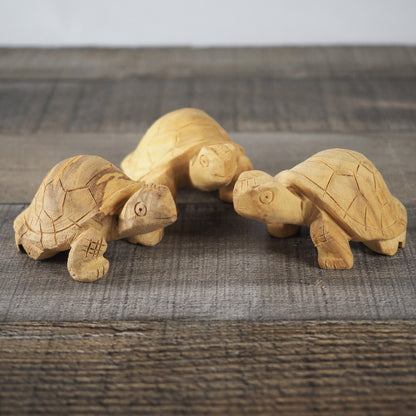The image depicts three intricately hand-carved wooden turtles arranged in a triangular formation on a dark gray wooden table. The turtles, varying in shades of light brown wood, appear to interact with each other; the one on the right faces left, the one on the left faces right, and the center turtle looks towards the one on the right. Each turtle's shell features carefully etched patterns of crevices and grooves, extending to detailed carvings on their knees and foreheads. Their faces, adorned with small, round eyes and subtle smiles, give them a lifelike and endearing appearance. Measuring approximately three to four inches tall and five to six inches long, these smaller-than-life turtles sit on a table that has visible wood grains and a blue wall backdrop, enhancing the overall homely and artistic setting of the picture.